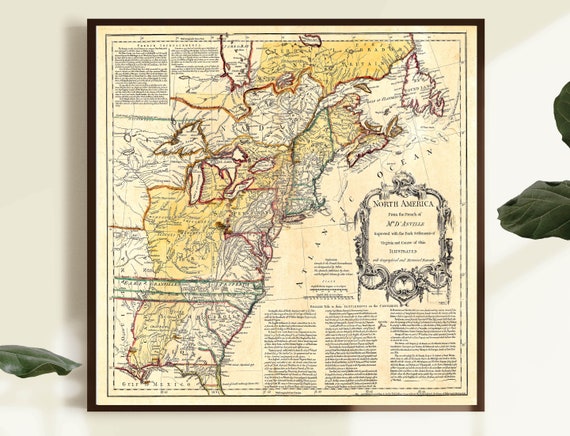The image depicts a vintage-style map of North America, prominently displaying the eastern portions of the United States and parts of Canada. The map, which features a dark yellow background typical of aged paper, is framed in a dark brown frame against a cream-colored wall. The title "North America" is prominently visible alongside "Atlantic Ocean." The map includes sections highlighted in green, yellow, and red, but the shapes do not correspond to modern-day state borders. Textual details on the map are present but not legible. The scene is complemented by greenery, with two dark green plant leaves entering from the right and one from the left, casting natural shadows on the wall behind the map. The map appears to be part of a styled display, possibly for an Etsy store, where elements like shadows and leaf veins are noticeable, suggesting a deliberate and artistic arrangement.